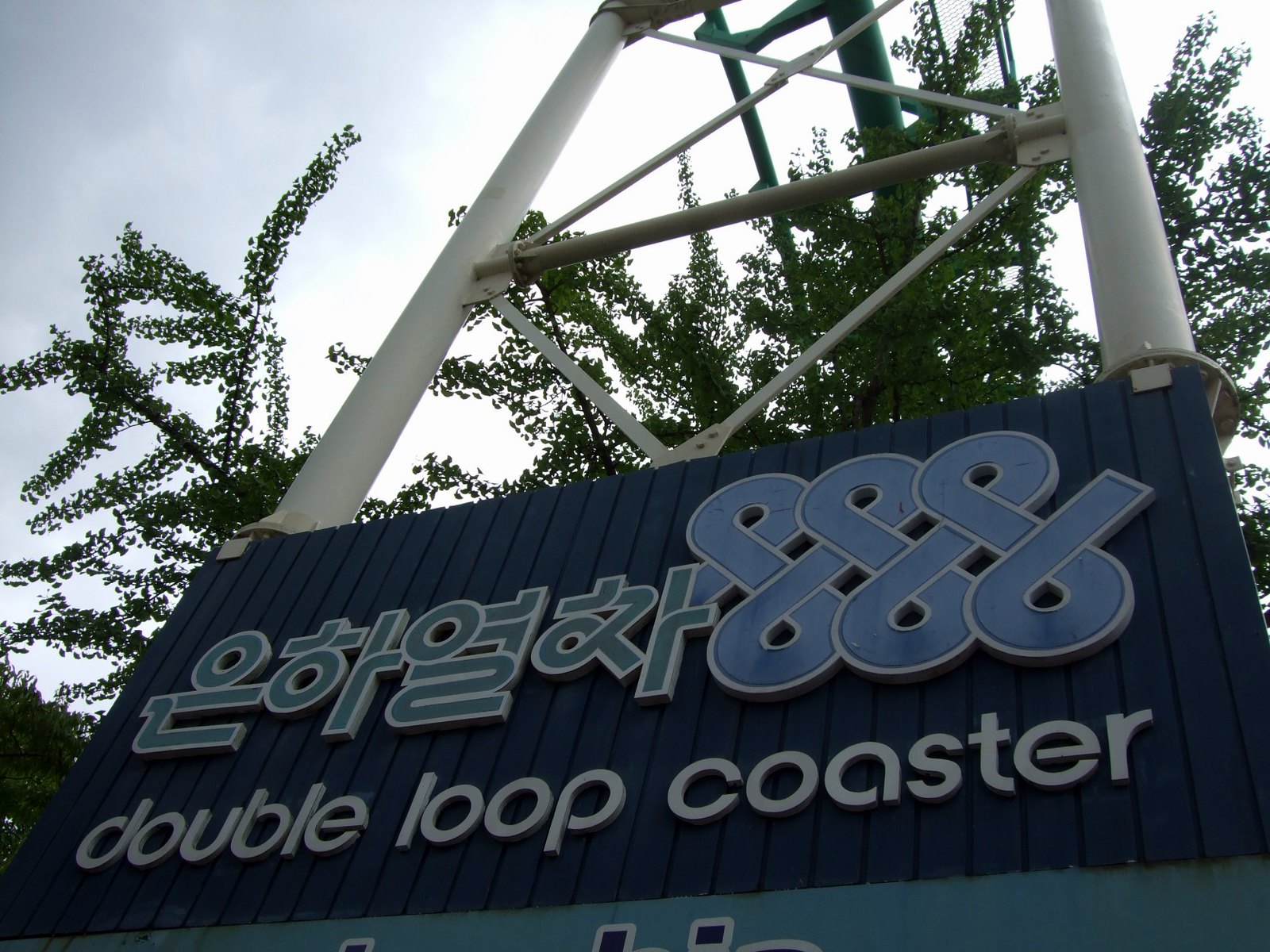The image presents a detailed upshot of a roller coaster sign at an amusement park. The sign, centrally placed, boasts a dark blue background with Korean characters in green, outlined in white on the left. Adjacent to the Korean text are three intertwined, infinity-like, looped symbols in blue with white outlines. The text "Double Loop Coaster" is displayed in modern, white sans-serif font beneath the symbols, with an unreadable green banner below. The sign consists of multiple dark blue wooden planks aligned vertically, supported by metal pipes and bars likely part of the structure that holds the coaster tracks, visible in green metal above. Surrounding the sign, bushy trees with tiny leaves reach into the frame, blending with the metal framework. The sky is cloudy and gray, with light gray clouds particularly on the left, casting a muted, overcast light over the entire scene.